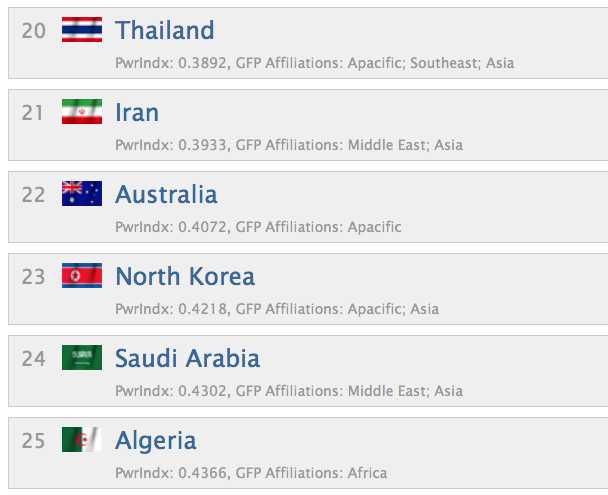This screenshot displays a series of flags representing different nations, each accompanied by their respective Power Index (PWR index) and geopolitical affiliations. The information is presented in a gray rectangular area, listing the countries numerically from 20 to 25 as follows:

1. **Number 20: Thailand**
   - **Flag**: Thailand
   - **Power Index (PWR index)**: 0.3892
   - **Global Firepower (GFP) Affiliations**: Pacific Southeast Asia

2. **Number 21: Iran**
   - **Flag**: Iran
   - **Power Index (PWR index)**: 0.3933
   - **Global Firepower (GFP) Affiliations**: Middle East and Asia

3. **Number 22: Australia**
   - **Flag**: Australia
   - **Power Index (PWR index)**: 0.4072
   - **Global Firepower (GFP) Affiliations**: Pacific

4. **Number 23: North Korea**
   - **Flag**: North Korea
   - **Power Index (PWR index)**: 0.4218
   - **Global Firepower (GFP) Affiliations**: Pacific and Asia

5. **Number 24: Saudi Arabia**
   - **Flag**: Saudi Arabia
   - **Power Index (PWR index)**: 0.4302
   - **Global Firepower (GFP) Affiliations**: Middle East and Asia

6. **Number 25: Algeria**
   - **Flag**: Algeria
   - **Power Index (PWR index)**: 0.4366
   - **Global Firepower (GFP) Affiliations**: Africa